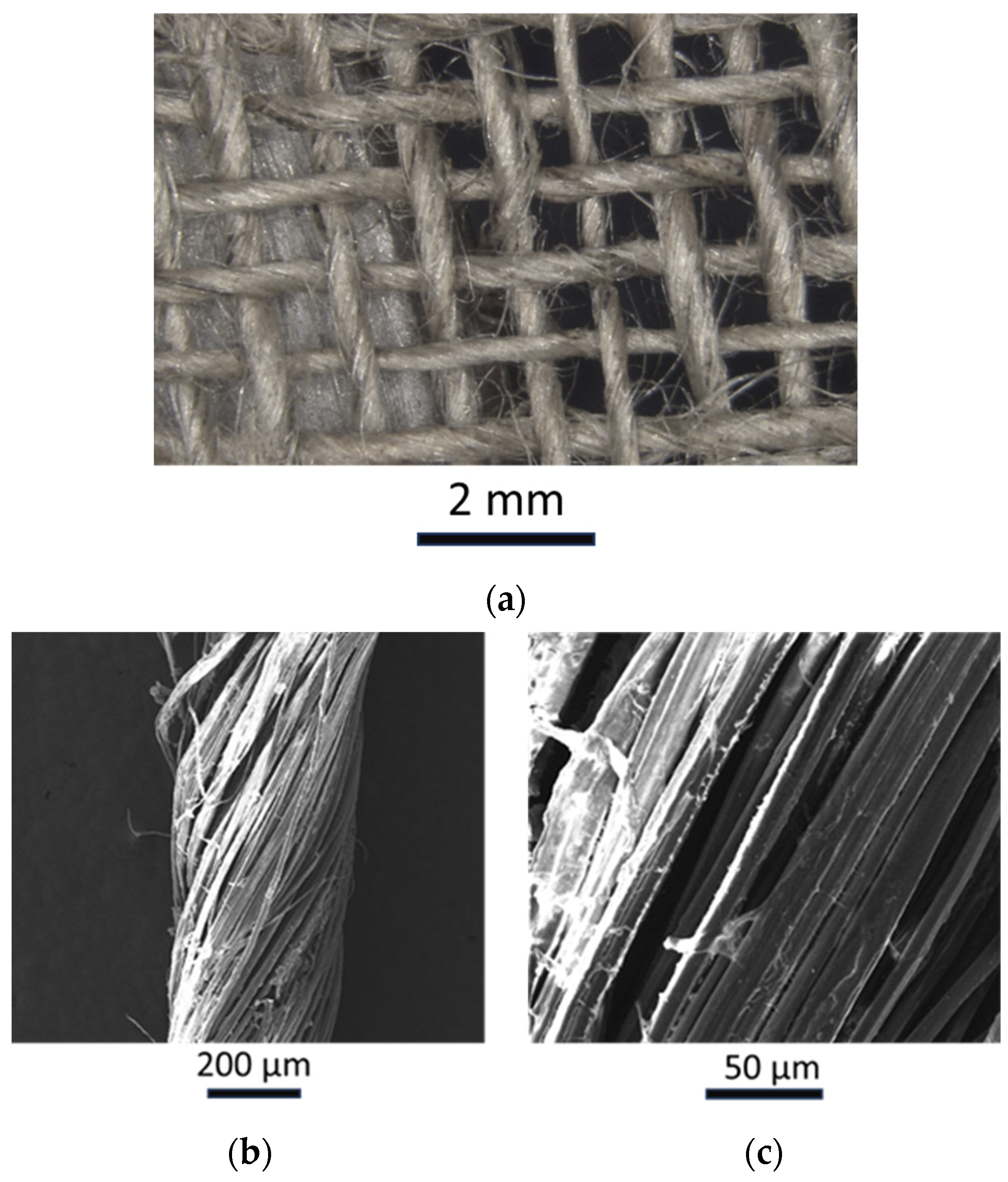This scientific image display consists of three distinct pictures showcasing fibers from a woven basket through various magnifications. The top image is a color photograph depicting a woven basket made from what appears to be burlap string. The basket has an over-under weaving pattern, and a wooden board is placed inside, adding structure. Below this image, the text "2mm" is visible along with a label "A" in parentheses.

In the lower left-hand corner, the first black-and-white image labeled "B" (with "200μm" denoted beneath it) presents a close-up view of the fibers through an electron microscope. This vertical shot reveals the fibers' twist and stretch along the length of the basket, highlighting their intricate striations and structural details.

The bottom right image, marked "C" with "50μm" indicated underneath, offers an even closer magnification. This extreme close-up shows the hemp fibers in meticulous detail, revealing their scruffy, split texture and almost square-like appearance when viewed at this high level of magnification.